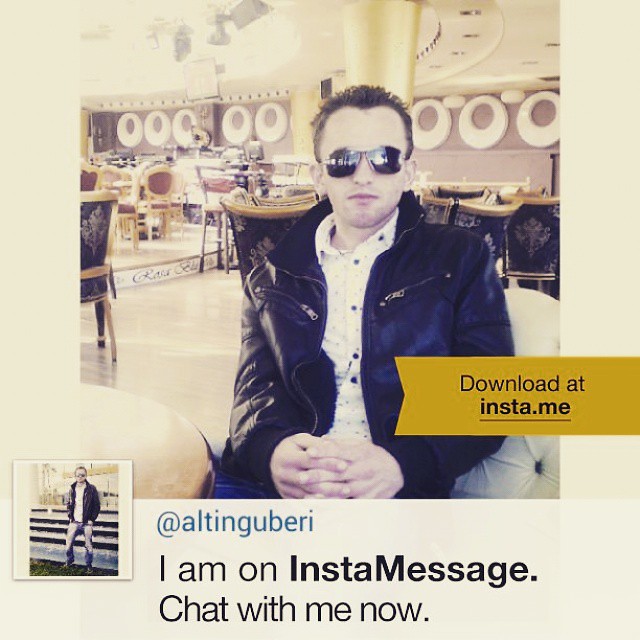The image features a man named Alton Guberi, who is sitting in what appears to be a large, empty restaurant or food court with various tables and chairs scattered behind him. The background wall is a pinkish hue with horizontal white circles. Alton is seated in a chair, wearing a black leather jacket with zippers above both breasts, a white shirt with buttons on the left side, and dark sunglasses. His brown spiky hair reveals a prominent forehead, and his hands are clasped in his lap. He has an expressionless face. In the bottom left corner of the image, there is a smaller thumbnail of Alton, dressed in the same leather jacket, white shirt, and dungarees, standing against a fence. The image includes promotional text with a yellow mustard banner on the left side that says "Download at insta.me" and "I am on InstaMessage. Chat with me now." The entire setup of the image, including the green bar and light blue framing, gives the impression of an online profile or advertisement, possibly for a dating app or social media platform.